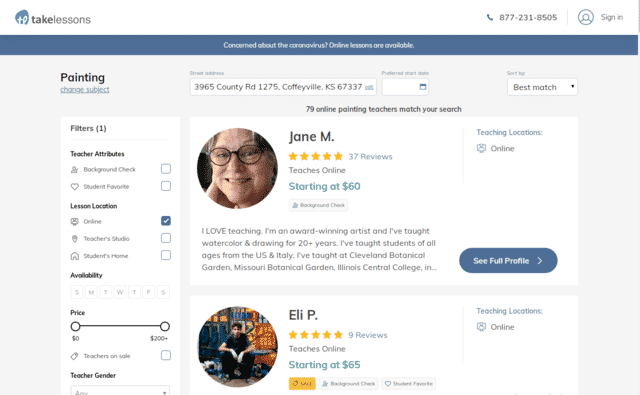At the top of the image, there is a white border approximately an inch thick. On the left side of this border, there is a small blue circle containing the lowercase letters "t" and "l." To the right, in bold black text, is the word "Take," followed by the less bold, black word "Lessons." On the right side of the border, there is the text "Sign In," accompanied by a circle with a profile icon inside it. To the left of this circle is a phone icon followed by a phone number.

Approximately half an inch below this border, there is a dark blue strip with white text in the center that reads, "Concerned about the coronavirus? Online lessons are available."

The area below this strip has a light blueish-gray background. About an inch in from the left side, at the top, is the bold black word "Painting," followed by the words "Change Subject" beneath it. Below that, there's a small white rectangle; at the top left of this rectangle, the word "Filters" is written, and to the right, it says "More." 

Underneath this, the text reads "Teacher Attributes" with two related options listed below. Next, there's a section titled "Lesson Location" with three location-related options. Under that is the "Availability" section with the days of the week abbreviated (SMTWTFS). Below this, there's a price range filter ranging from $0 to $200. The final visible section is labeled "Teacher Gender," but it extends off the bottom of the page, making it unreadable.

On the right side of the image, there is a search bar where users can enter a street address. Adjacent to the search bar is a square containing a calendar and some text that is not clear. To the right of the calendar, there is a drop-down menu labeled "Best Match." 

At the center of the page, the text indicates, "79 online painting teachers match your search." Below this, there are profiles of two teachers. Each profile displays the teacher's profile picture on the left, the teacher's name to the right, their star rating, number of reviews, the mode of lesson delivery (e.g., online), and the price of lessons. Additional information about each teacher is listed below their names.